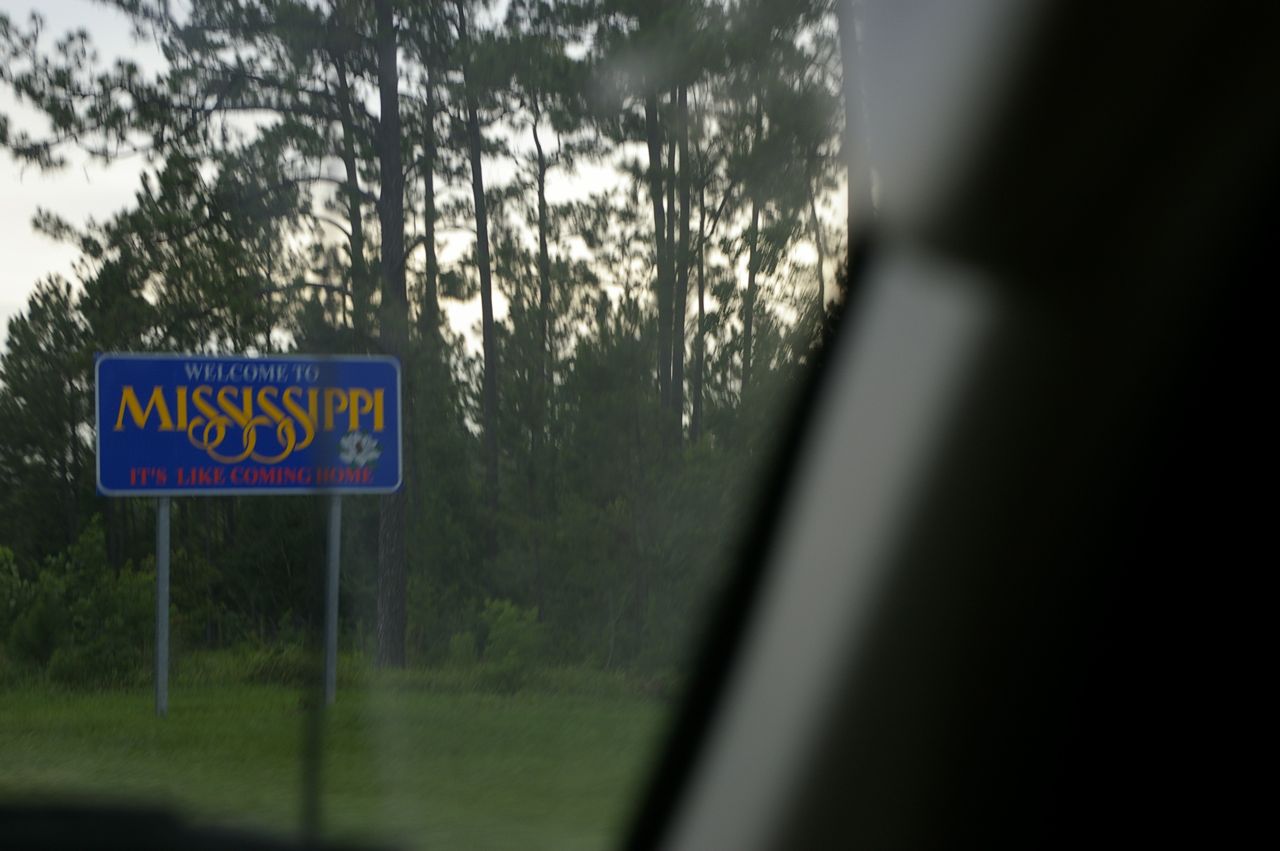The photograph captures an outdoor scene shot from inside a vehicle, presumably while in motion. The interior frame of the passenger side door and a closed window are visible in the foreground, indicating that the person taking the picture is seated in the front passenger seat. The focus of the image is a blue highway sign with white, gold, and red lettering that reads "Welcome to Mississippi." The text "Welcome to" is in white, "Mississippi" is in gold, and "It's like coming home" is in red. A small white flower adorns the bottom of the second 'P' in "Mississippi." The backdrop of the scene features a gray, overcast sky, tall green-leaved trees, and a grassy area where the sign is installed.